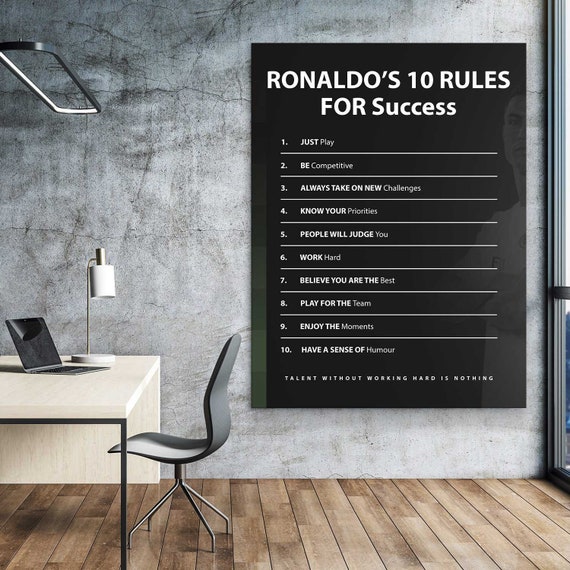This vertical photograph captures a sleek, contemporary office space with an air of minimalism and motivation. The setting features a medium brown plank laminate floor and a modern distressed wall with a subtle black-and-white hazy design. Dominating the right side of the image is a large, black rectangular poster hanging on the wall, titled in bold white capital letters, "RINALDO'S TEN RULES FOR SUCCESS." Beneath the title, the rules are numbered one to ten, each with specific words capitalized: 

1. JUST PLAY
2. BE COMPETITIVE
3. ALWAYS TAKE ON NEW CHALLENGES
4. KNOW YOUR PRIORITIES
5. PEOPLE WILL JUDGE YOU
6. WORK HARD
7. BELIEVE YOU ARE THE BEST
8. PLAY FOR THE TEAM
9. ENJOY THE MOMENTS
10. HAVE A SENSE OF HUMOR

The poster's final line reads, "TALENT WITHOUT WORKING HARD IS NOTHING," all in capital letters. A faded image of Cristiano Ronaldo with crossed arms serves as the backdrop. Below the poster, a sleek white wooden desk is situated, featuring a metal desk lamp with a white shade and an open Mac laptop positioned to the right. The desk is paired with a sleek black chair characterized by its simplicity and functionality, with a metal frame and no cushion. Completing the office ambiance is an oval-shaped metal ceiling lamp hanging above the desk. The photo exudes a mock-up office feel, with objects seemingly superimposed, contributing to the overall modern and motivational aesthetic.